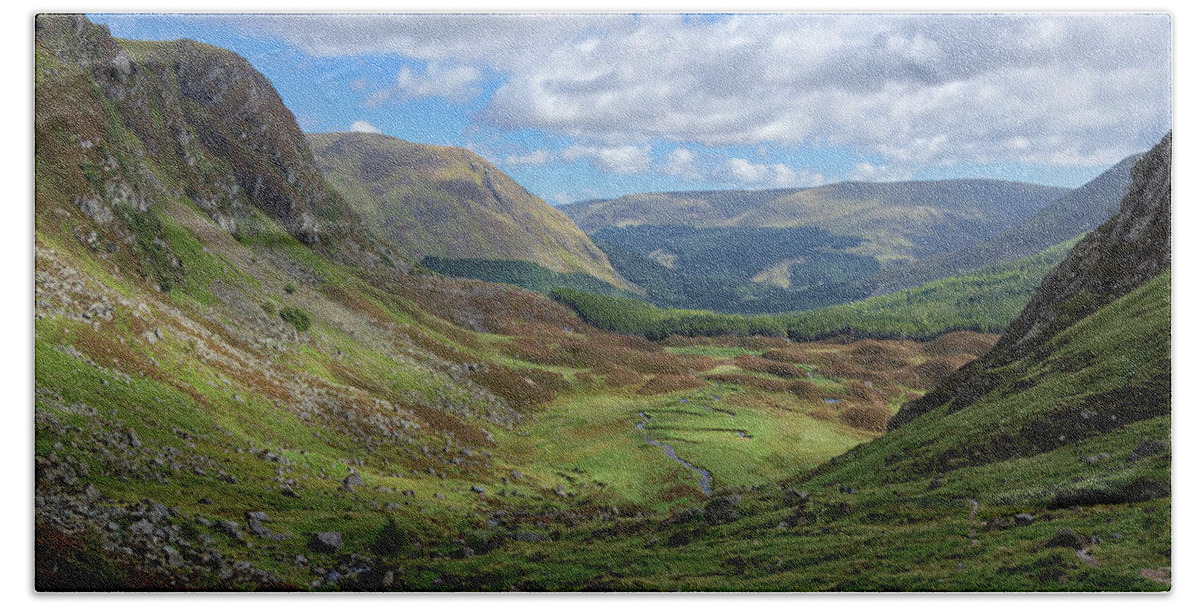The image is a realistic depiction, possibly a photograph, of a very green valley nestled between sloped mountains or hills, reminiscent of the Scottish Highlands. The valley is characterized by a tiny, winding creek or stream running down its middle, with a sweeping vista uninhabited by any living beings. The scene is predominantly lush and green, though there are patches of brown suggesting dry leaves or less vegetated areas. Grayish stones and rocks are also scattered throughout the foreground.

The sky is a mix of white clouds and pockets of blue, with clouds rolling in from the right side and some gray hues hinting at more overcast conditions. The clouds dominate much of the sky but allow glimpses of blue to peek through. The left side of the image features a taller cliffside extending upward. The entire landscape fosters a sense of serene, natural beauty with the subtle grainy quality of the picture adding a somewhat painted, yet lifelike, texture.